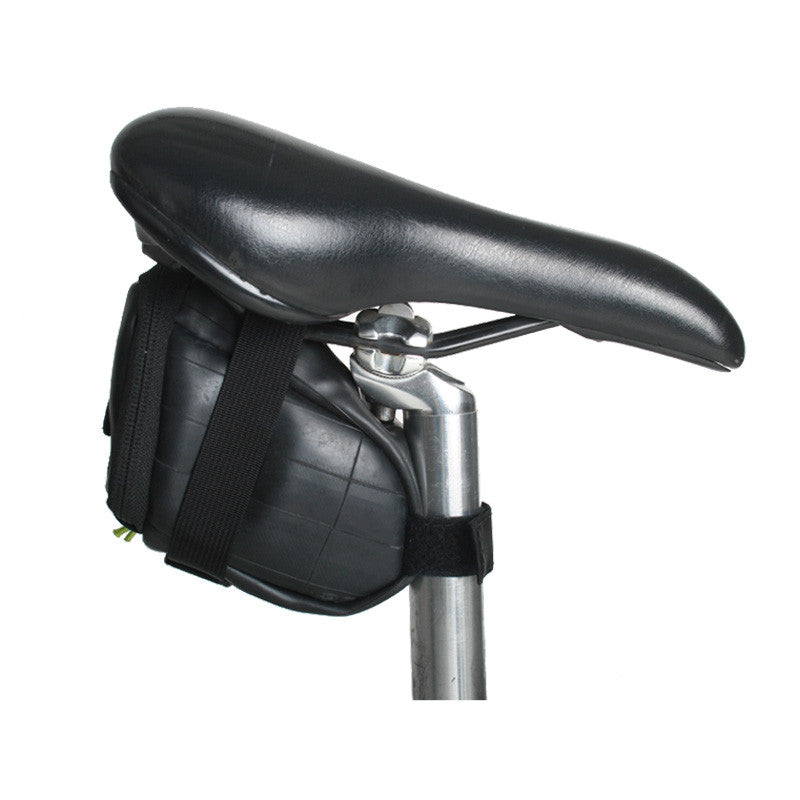The photograph showcases a black bicycle seat set against a white background. The seat is prominently displayed from the side, catching glimmers of light along its sleek surface. It is mounted on a silver metal pole, which is integral for attaching the seat to a bicycle. Affixed beneath the seat is a black leather pouch that is also reflective and features lined detailing on its side. The pouch is securely fastened to both the seat and the metal pole using black Velcro straps, with one strap looping through the metal connector of the seat and another securing the pouch to the pole itself.